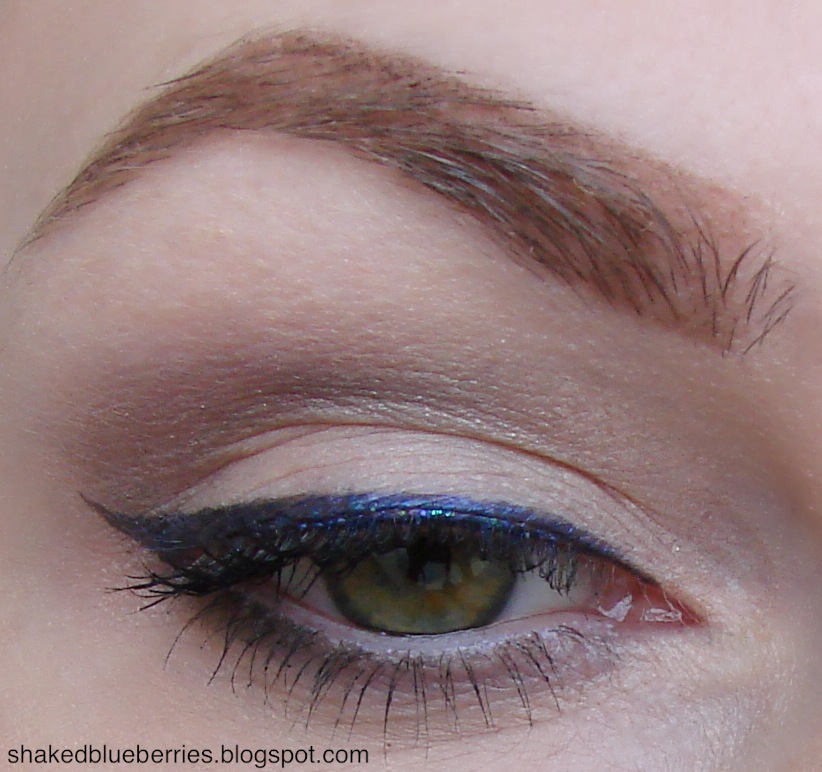This image is an extremely close-up shot of a woman's right eye, showcasing intricate makeup. The iris of her eye is primarily brown with a hint of light blue at the center, and she has green eyes overall. Her eyebrow above the eye is carefully manicured into an arched shape, filled in with a brown eyebrow pencil, complemented by softer, lighter brown makeup behind it. There is a shimmering tan eyeshadow that blends up towards her eyebrow. Over her top eyelid, she wears a striking, bright blue eyeliner that extends outward in a dramatic, cat-eye fashion, transitioning into a smoky eye effect toward the outer corner. The eye makeup is completed with black mascara accentuating her very long eyelashes. On the lower left corner of the image, there are small black letters against her pale skin tone, reading "shakedblueberries.blogspot.com." The overall color palette of the photo incorporates flesh tones with vibrant and smoky hues, capturing the elaborate detail of the makeup.